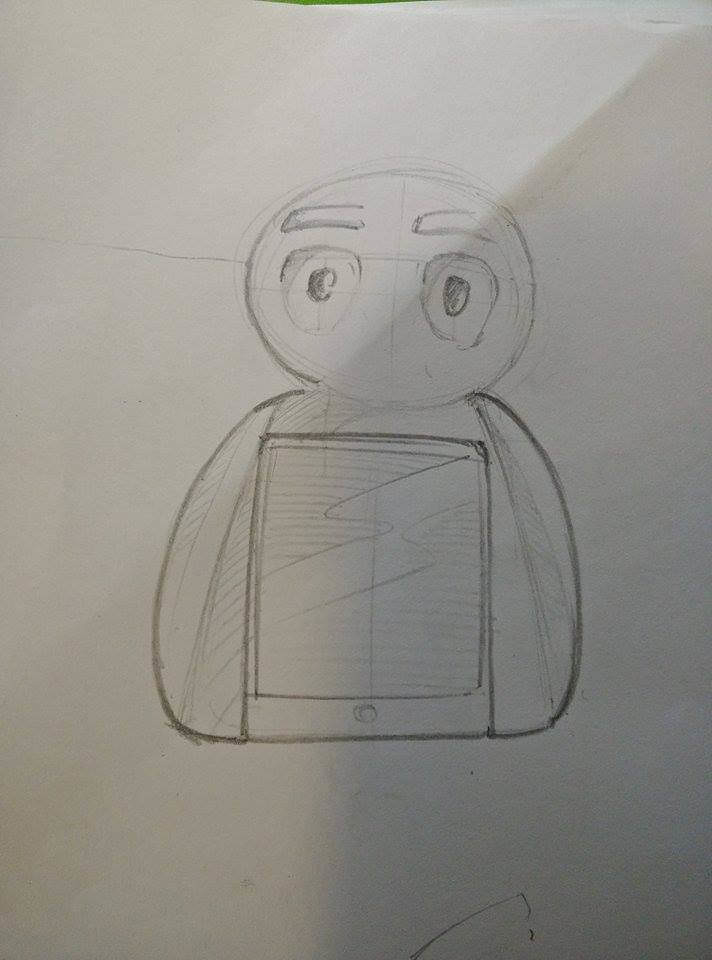This image showcases a hand-drawn pencil sketch on a white sheet of paper, depicting an endearing, stylized character. The character has a disproportionately large head, devoid of a mouth or nose but adorned with thick eyebrows and large, irregularly-sized pupils. The drawing appears to contain numerous eraser marks, suggesting the artist made several corrections during the creation process. Despite some unintended lines across the face, the character's expressive eyes stand out. The figure's arms hang straight down without defined hands, and slight shading accentuates their form. A boxed element is present on the character's chest, partially shaded at the top and bottom. Notably, the character features a distinct belly button, but lacks a discernible body or hands. The composition is completed by a scribbled line at the bottom which appears accidental, rising and falling in a random fashion.